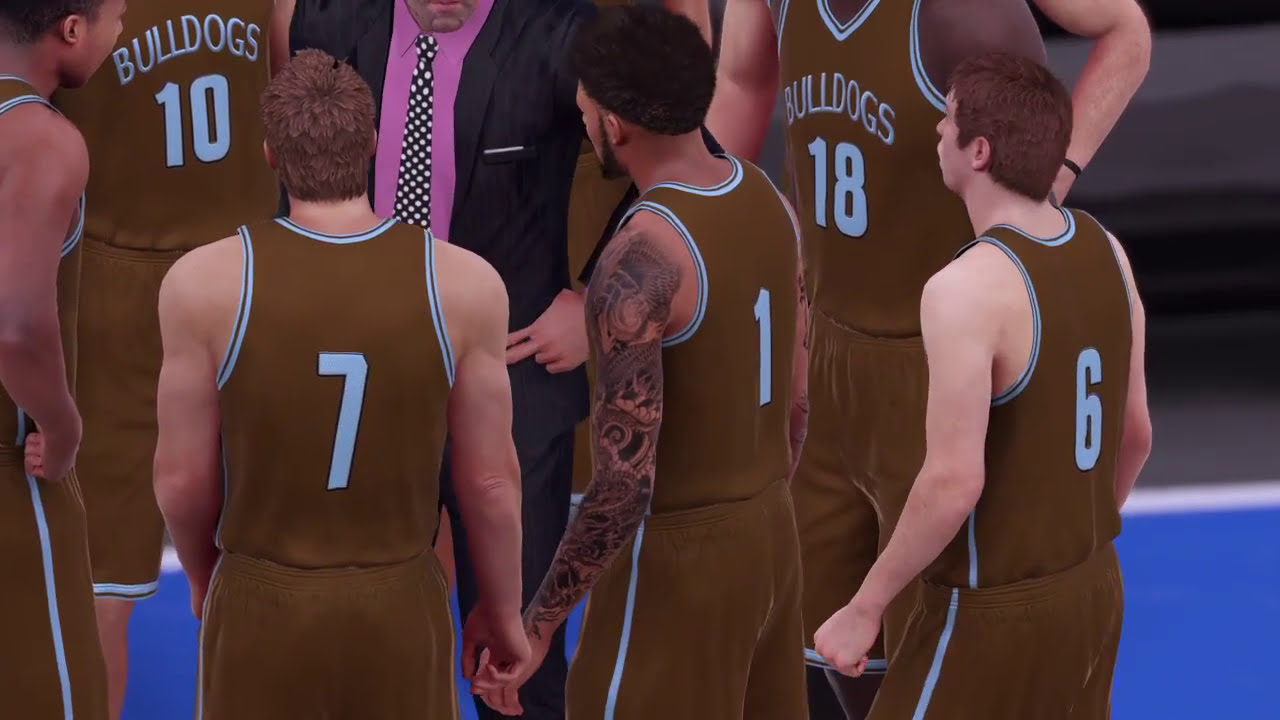The image appears to be a screenshot from a basketball video game, characterized by decent but not photorealistic graphics, rendering it somewhat cartoonish. The scene takes place on a blue-painted basketball court with visible bleachers in the background. At the center, a group of basketball players huddles around their coach. The players, wearing brown jerseys with white trimming and the team name "Bulldogs" emblazoned on the front, display various jersey numbers including 10, 7, 1, 18, and 6. The central player, who appears to be African American with a full sleeve tattoo, draws focused attention from his teammates. Among them, two are Caucasian and another African American player is visible, donning the number 18 jersey. The coach, partially cropped out, is attired in a distinctive black suit, pink shirt, and a black and white polka dot tie. The collective gaze of the players suggests attentiveness to the coach’s instructions.